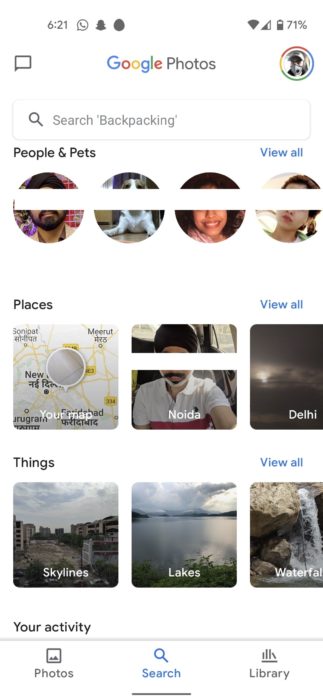A detailed view of the Google Photos interface is displayed, presenting a clean, white-themed design. At the top of the screen, the time is shown as 6:21 AM on the left side, accompanied by a phone icon within a speech bubble, and several other icons. On the top right, the battery icon indicates a 71% charge, and below it, there's a profile picture encapsulated in a circle with Google’s characteristic colors. 

Directly underneath is a search field labeled "Search backpacking", followed by a section titled "People & Pets". This section invites the user to "View All" and displays four circular thumbnails representing three people and one dog.

Further down, a "Places" section includes a "View All" option and displays three categories: "Your Map" on the left with a map thumbnail, "Noida" in the center with a partially obscured photo of a person, and "Delhi" on the right showing a gray sky. 

Below, the "Things" section also offers a "View All" option and showcases three thumbnails labeled "Skylines," depicting a cityscape, "Lakes," showing a lake, and "Waterfalls," displaying a waterfall.

At the bottom, the interface features the "Your Activity" section, highlighting three options: Photos, Search, and Library, inviting the user to explore their captured memories and searches.